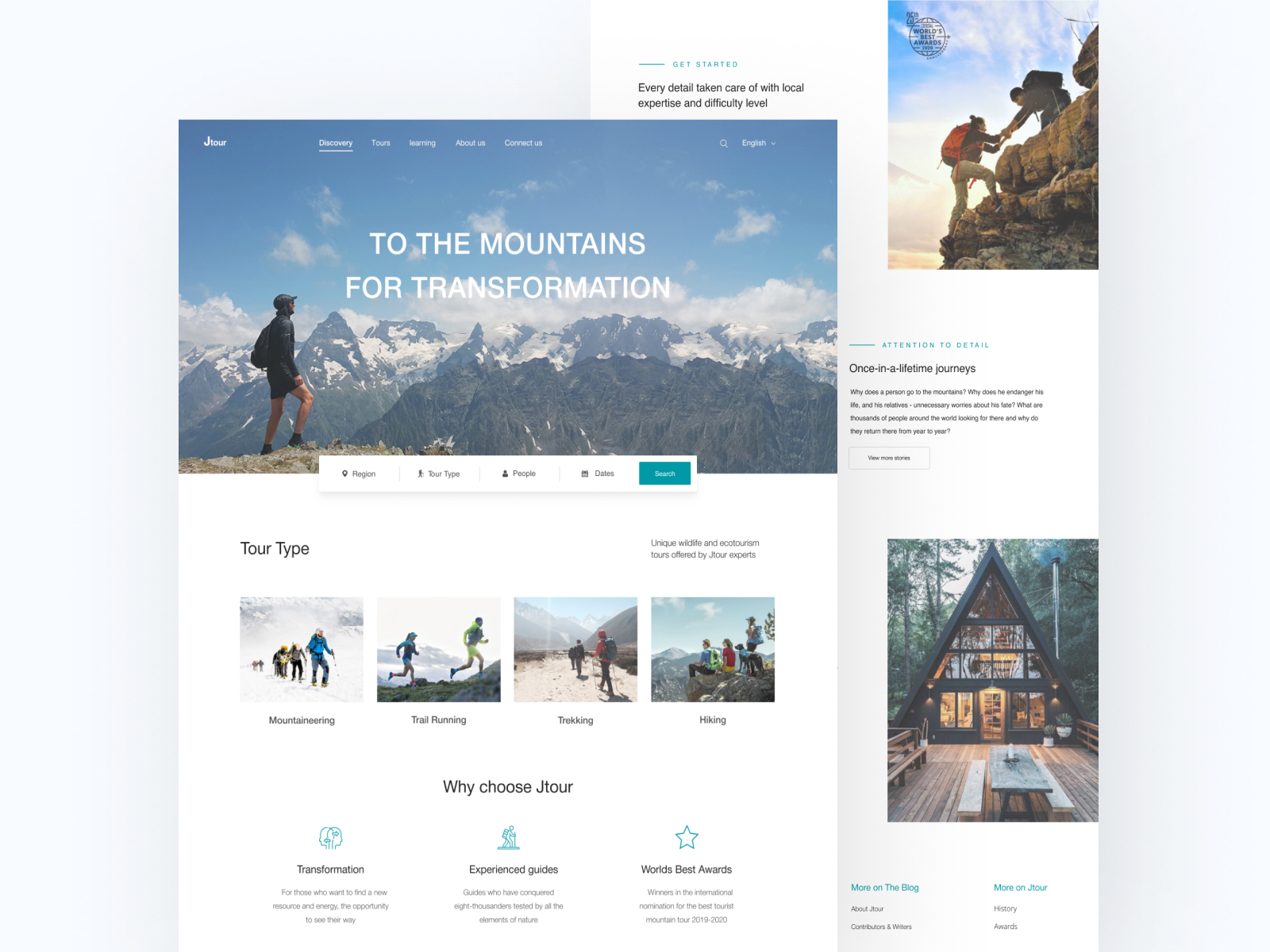The image depicts the homepage of a website called JTour, dedicated to enthusiasts of mountaineering and related outdoor activities. The website offers four main types of adventures: mountaineering, trail running, trekking, and hiking. The homepage is dominated by a striking photograph of a man standing near a mountain summit, gazing out at a breathtaking, cloud-filled landscape. The central focus of the image features a motivational tagline: "To the mountains for transformation." 

In the top left corner, the JTour logo is prominently displayed, while the top right corner includes options for changing the website's language and a search function. Each of the four adventure categories is represented by distinct icons and images. Below this, a detailed section explains why JTour is the preferred choice for outdoor enthusiasts, emphasizing three core values: Transformation, Experienced Guides, and World's Best Awards. 

On the right-hand side of the screen, additional dramatic photographs showcase potential destinations and accommodations, designed to capture the viewer's imagination and entice them into planning their next adventure with JTour.